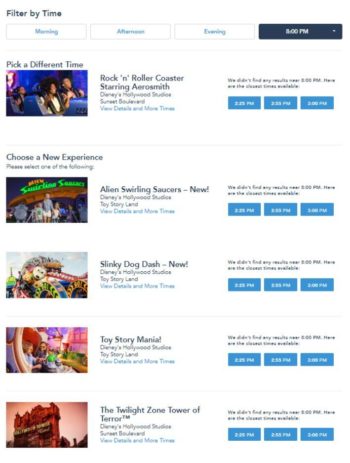This screenshot displays the schedule for five distinct experiences at Disney's Hollywood Studios. Each experience is neatly presented on a separate line, divided by faint gray lines for clarity. Every listing includes a thumbnail image on the left, a brief description in the center, and the available starting times to the far right. 

1. **Rock 'n' Roller Coaster Starring Aerosmith**: Located in Sunset Boulevard, Disney's Hollywood Studios.
2. **Alien Swirling Saucers-New**: Situated in Toy Story Land within Disney's Hollywood Studios.
3. **Slinky Dog Dash-New**: Also found in Toy Story Land, Disney's Hollywood Studios.
4. **Toy Story Mania**: A popular attraction in Toy Story Land, Disney's Hollywood Studios.
5. **The Twilight Zone Tower of Terror™**: Another exciting experience located in Sunset Boulevard, Disney's Hollywood Studios.

Each of these attractions is meticulously listed to enhance the user’s ability to plan their visit efficiently.